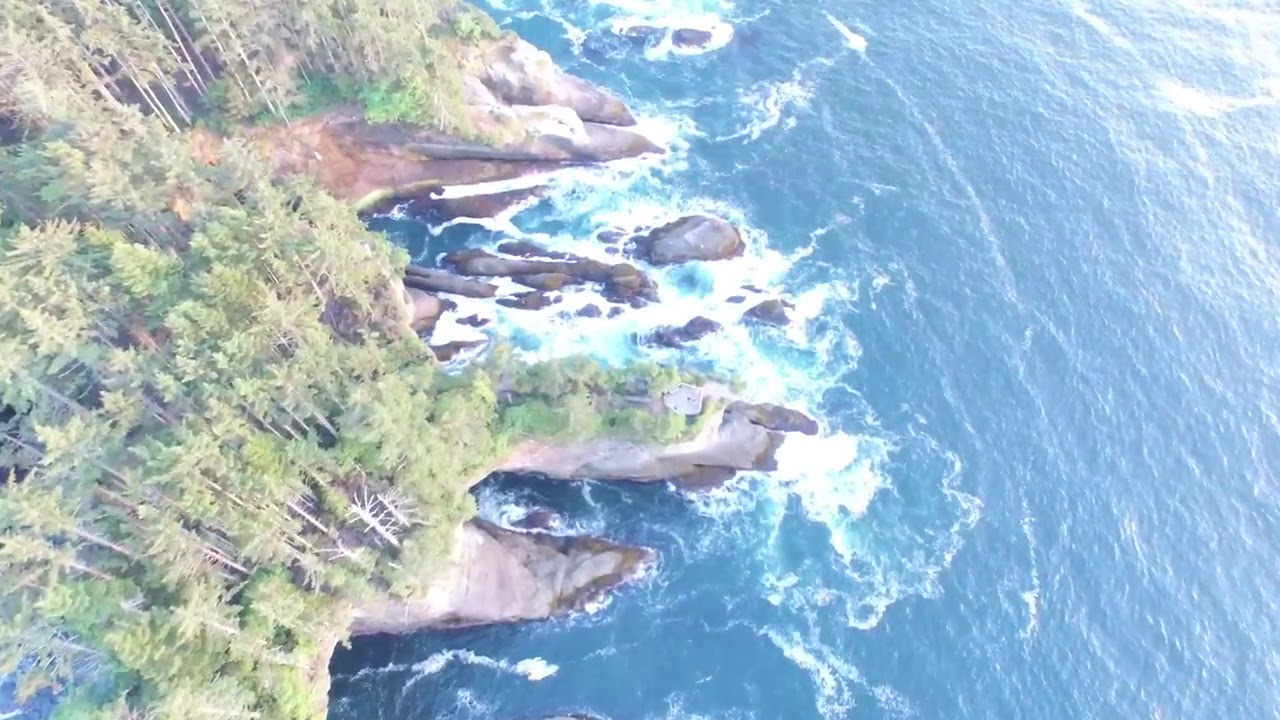The image is an aerial, top-down photograph of a large, possibly northern body of water that could be an ocean or an extensive lake. The water exhibits a striking blue hue with small waves crashing against large, round, gray, white, and brown rocks, creating white splashes. Centrally located in the image is a rocky outcrop where the waves are most prominent. There is a pentagon-shaped viewpoint built on one of the jagged rocks protruding into the water, connected to the mainland by a walkway. This platform extends inland, leading to a dense forest of tall, slender pine trees, approximately 30-40 feet in height but only around 8 feet wide. The forest's edge is directly adjacent to the rocky coastline, with little to no sandy or dirt separation. On the right side of the image, vast, uninterrupted water dominates the scene, while the left side showcases the repetitive pattern of narrow pine trees with minimal undergrowth. The coastline features numerous jutting points and small inlets, where the light blue water forms caverns and waterways between the craggy rocks. A few people are visible on the pentagon-shaped outlook, adding a sense of scale and human presence to this rugged, scenic landscape.